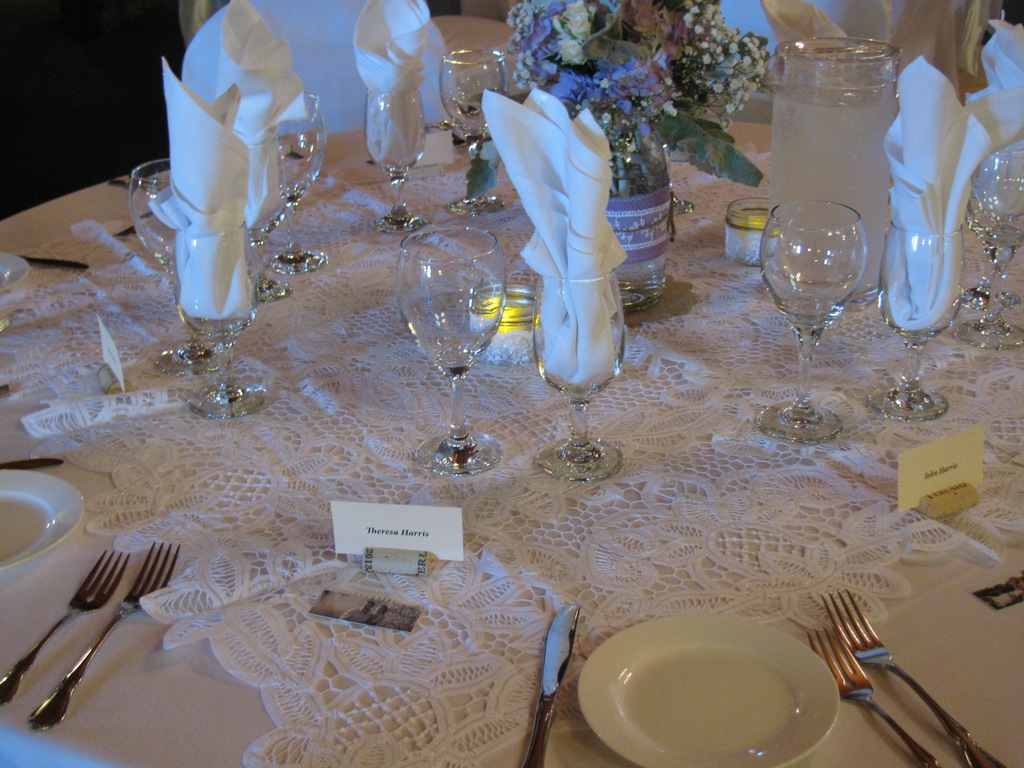This image captures an elegant, wedding reception table meticulously set for five guests. The table is draped with a white circular tablecloth, overlaid with a large, square, white lace doily featuring intricate floral designs. At each setting, there's a white ceramic plate accompanied by two forks placed to the left and a knife to the right. Surrounding the plates, there are pairs of clear wine and water glasses, some of which have neatly rolled white napkins inside. In the center, a striking floral arrangement consists of purple and white-pink flowers with lush green leaves, housed in a clear vase wrapped with purple fabric. The table is adorned with small, circular candles and a large jug of water. Completing each setting are business card-sized white name cards, ensuring each guest's place is uniquely identified. The precise arrangement and lavish details suggest a formal and celebratory occasion, fitting for a wedding.